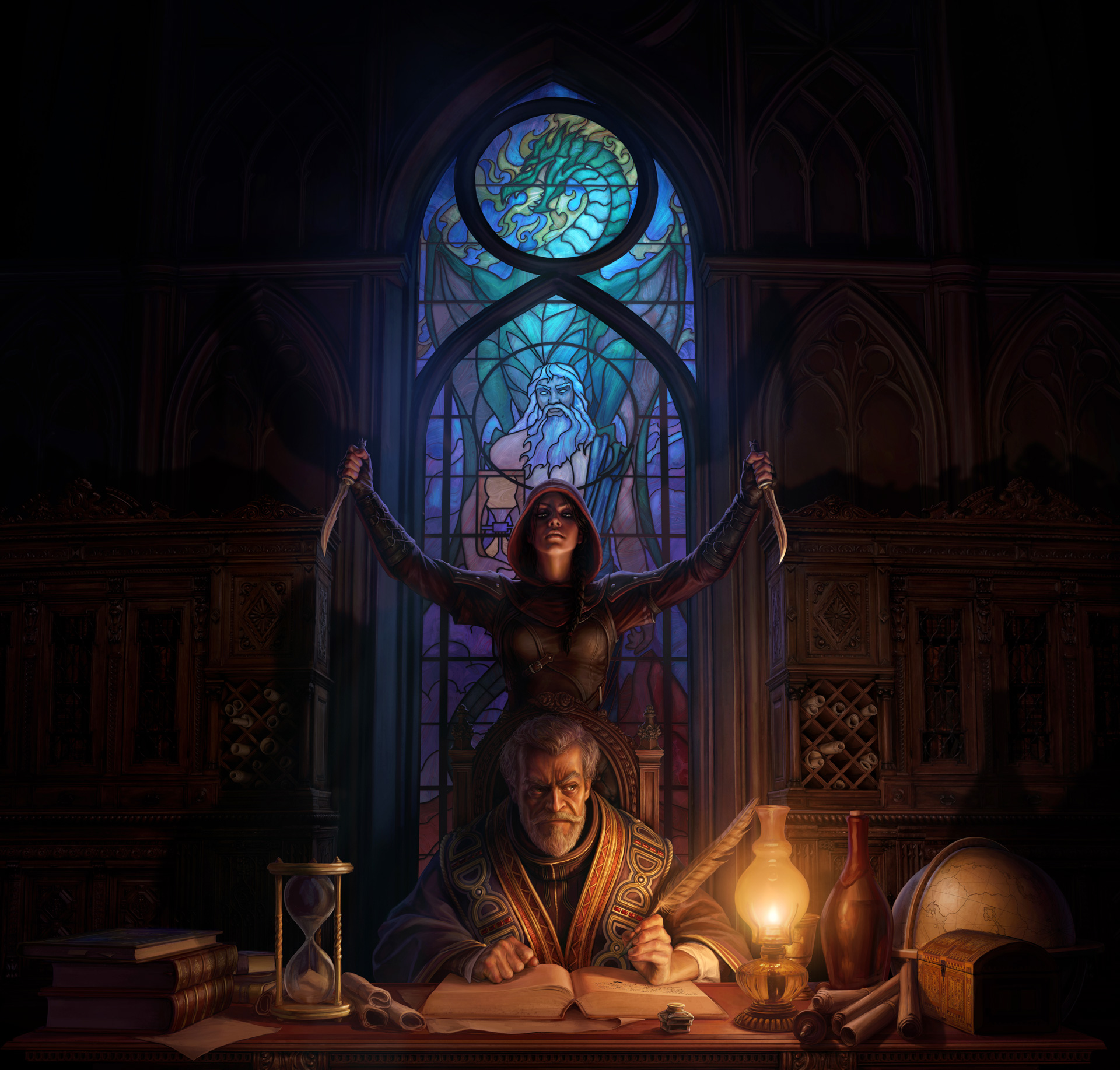The image portrays a meticulously detailed religious scene that appears to be a digitized piece or a painting—possibly watercolor or oil-based. At the center, a monk or priest is seated at a richly brown desk, dressed in ornate robes. He holds a feathered quill poised over a thick, open book, seemingly engrossed in writing. To his left, several books and an hourglass clock are displayed, while to his right, a yellow glass oil lamp casts a warm glow. On the table, there are also a vase and a globe, adding to the scholarly ambiance.

Behind the monk, a hooded woman clad in black or gray armor raises two large knives menacingly. Her presence looms over him suggestively, implying a potential attack, and the monk appears to be subtly aware of her, as his eyes dart to the side. The background is adorned with a stained-glass window featuring vibrant colors including green, yellow, blue, and purple, possibly depicting a dragon, which adds to the dramatic and enigmatic atmosphere of the scene. The carved paneling on the wall further accentuates the setting, placing the scene likely within a church or similar sacred space.